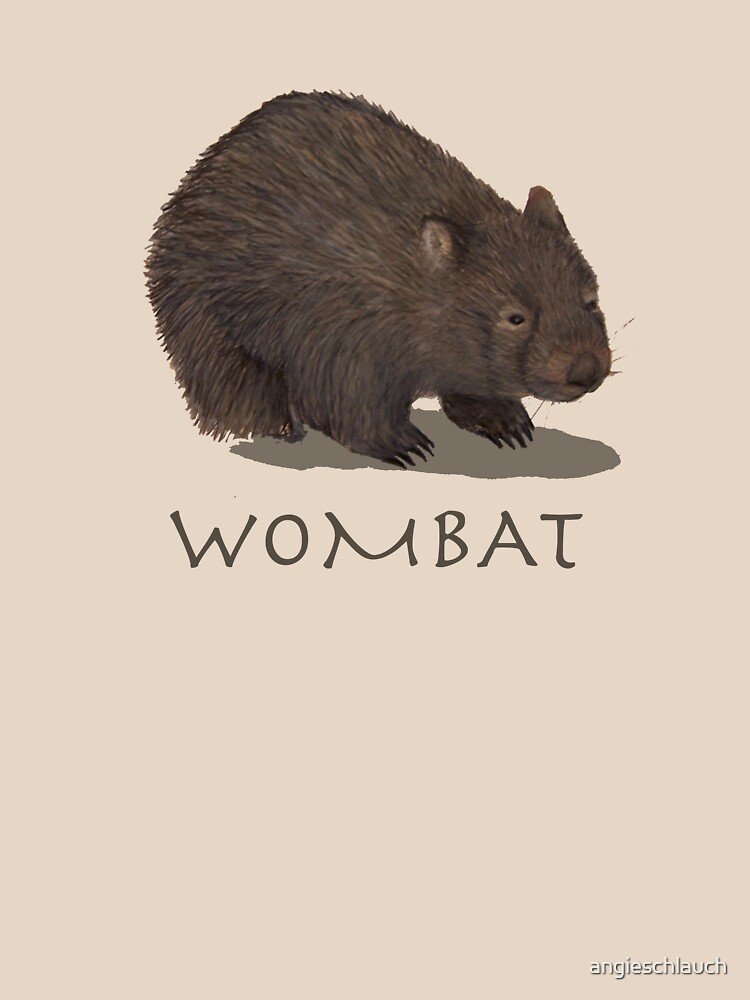This is a detailed and textured illustration of a wombat, immediately identifiable by the word "WOMBAT" displayed in all capital letters in modern stick print just below the animal. The wombat, depicted with brown fur and beady black eyes, looks like a small, bear-like creature with a snout, small ears, whiskers, and clear sharp claws. The illustration includes the wombat's shadow on a plain, pastel peach to light tan background. At the bottom, the words "Angie's Schlauch" (A-N-G-I-E S-C-H-L-A-U-C-H) are inscribed, suggesting perhaps the artist's attribution. The simplicity of the backdrop and the style of the illustration, hints that it might belong to a children's book, with its clean, uncluttered design emphasizing the charming character of the wombat itself.